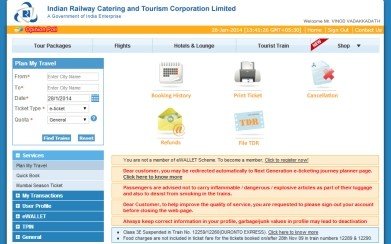The image features a bordered layout on both the left and right sides in medium blue. At the top left corner, a blue logo appears. The logo resembles a sideways triangle with curved lines extending from each point, and includes a blue square symbol with a white design in the middle. To the right of the logo, the text "Indian Railway Catering and Tourism Corporation Limited" is displayed in bold blue basic font. Below this, in non-bold blue text, it reads "A government of India" followed by an unreadable section due to low image quality.

On the right side of the image, the word "Welcome" is written in black. The overall image appears to be old and of low quality, making some details hard to decipher. Below this, an orange horizontal strip features an icon on the left and white text on the right with a fuzzy but thick red outline. Adjacent to this section, the date appears to read "26 Jan 2014," though it is difficult to make out clearly.

Further to the right are navigation options reading "Home," "Sign Out," and "Contact Us," each separated by white lines. Below these, additional menu tabs are divided by gray lines, with each tab appearing light blue and featuring a shiny central line for a 3D effect. The black text on these tabs reads "Tour Packages," "Flights," "Hotels," "Ensemble Lounge," "Tourist Train," and "Shop." Notably, the "Shop" tab has a small red banner in the top left corner with the word "New" in white text.